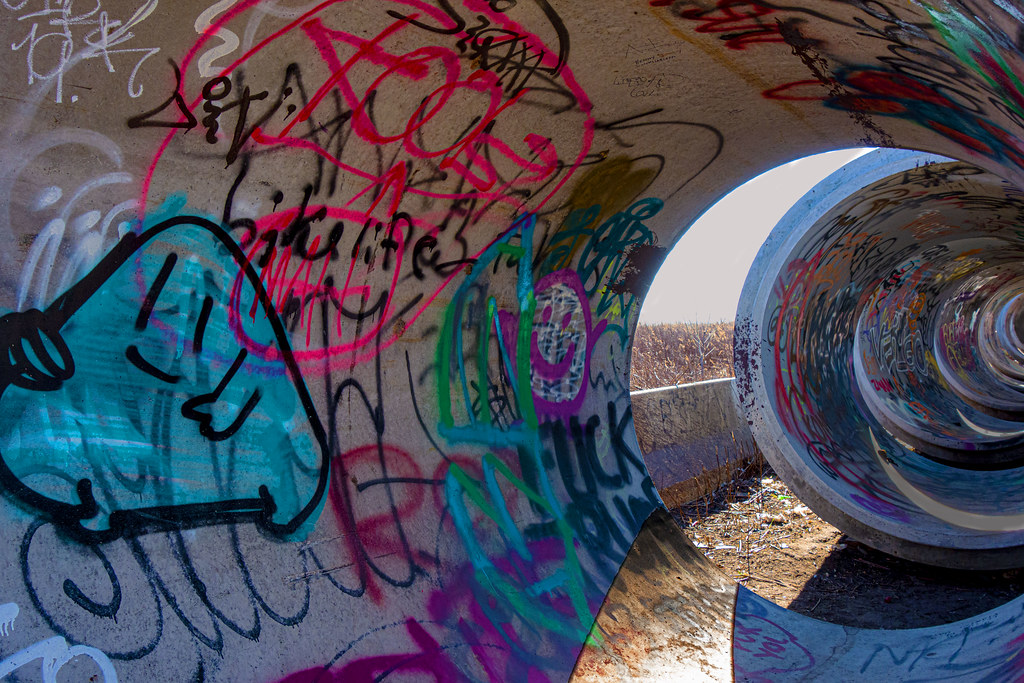The photograph captures the interior of a large, cylindrical concrete tunnel, heavily adorned with multicolored graffiti. The vantage point of the picture is from within one tunnel, looking out towards a series of similar, white pipes that create a seemingly endless, interconnected passageway. Daylight streams in from the end of the tunnel, revealing a brown field, dead grass, and a concrete barrier outside. The sky is a clear blue. Each tunnel, including the one in the foreground, is plastered with vibrant graffiti, featuring an array of colors such as pink, black, purple, and green. The graffiti includes various illegible scribbles, a blue ghost with a smiley face, and clearer phrases like "FUCK Trump" and "Maddie." Scattered among the grass outside the pipes is a discarded bottle, adding to the scene's abandoned feel.